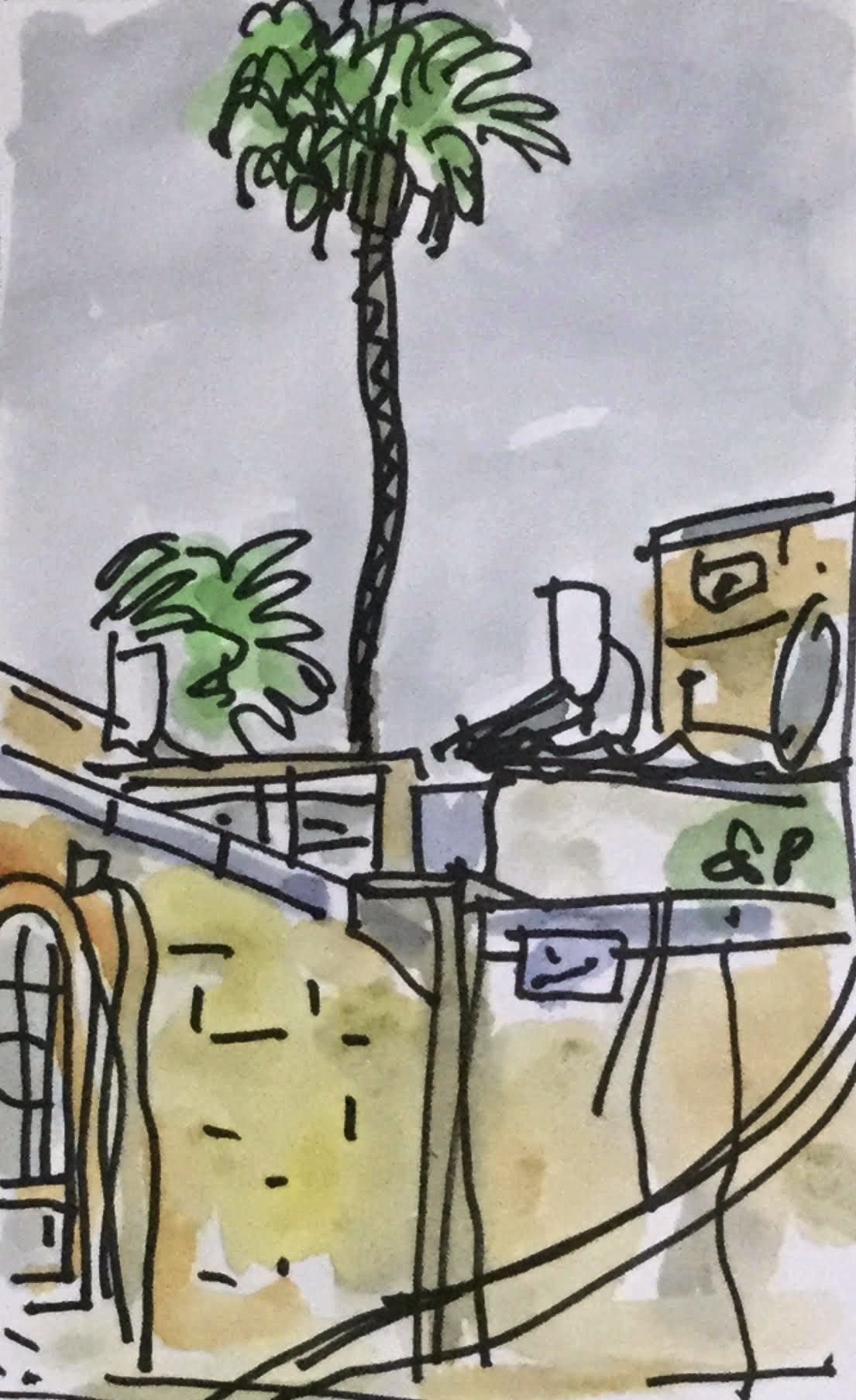This image appears to be a hand-drawn piece, initially outlined with a black marker and later enhanced with watercolor paints. The focal point of the artwork is a structure resembling a house, situated at the bottom of the scene. Prominently behind or above the house, a towering palm tree stretches upwards, with its leafy crown nearly touching the upper edge of the picture. 

To the left of the house, nestled near the base of the palm tree, a lush green bush adds a touch of verdancy. The house itself features a door with a distinct rounded top on the left side of the image, encircled by a gray border that also outlines the edges of the roof. The walls of the house are rendered in a tan hue, contributing to a warm and inviting atmosphere.

The sky above is painted in a gradient of light blue and purple, suggesting either dawn or dusk. Adding to the composition, a smaller, square building is positioned in the upper right corner, elevated above the house. The juxtaposition of these architectural elements against the vibrant natural features creates a balanced and visually appealing scene.